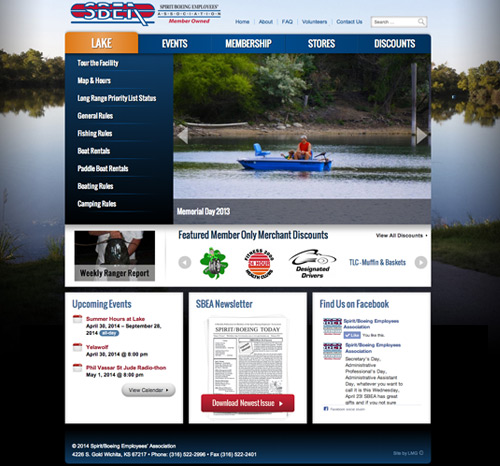The main page of the website is partially visible, focusing on the corners. The scene in the image includes trees, a body of water, and grass. The top section of the page features a mostly blue background with an orange rectangle at its start. 

Highlighted in white text are several categories:
- Lake
- Events
- Membership
- Stories
- Discounts

Further details include:
- "Tour of the facility"
- "Map"
- "Hours"
- "Long range"
- "Priority list status" (possibly)
- "General rules"
- "Fishing rules"
- "Best rentals"
- "Paddle boat rentals"
- "Boat enrolls"
- "Camping rules"

Prominently featured is an image showing two people in a small blue boat with a blue chair, set against a gray background. Below this image, in white text, is the caption "Memorial Day 2013," followed by a section titled "Feature" in blue, with subcategories including "Member Only," "Merchant Discounts," and "View All Discounts" in black.

Additional symbols are present, including a possible four-leaf clover and unknown fitness-related symbols in black. Text on the left side reads:
"Designated Drivers," with "TLC, Muffins, and Baskets" in blue text. There is a box on the left side listing "Upcoming Events," which mentions:
- Summerhouse at the Lake
- Yellow Wolf
- St. Jude (unspecified event)

Adjacent to this box is "SBA Newsletter" in blue, and the page also includes a "Find us on Facebook" link.